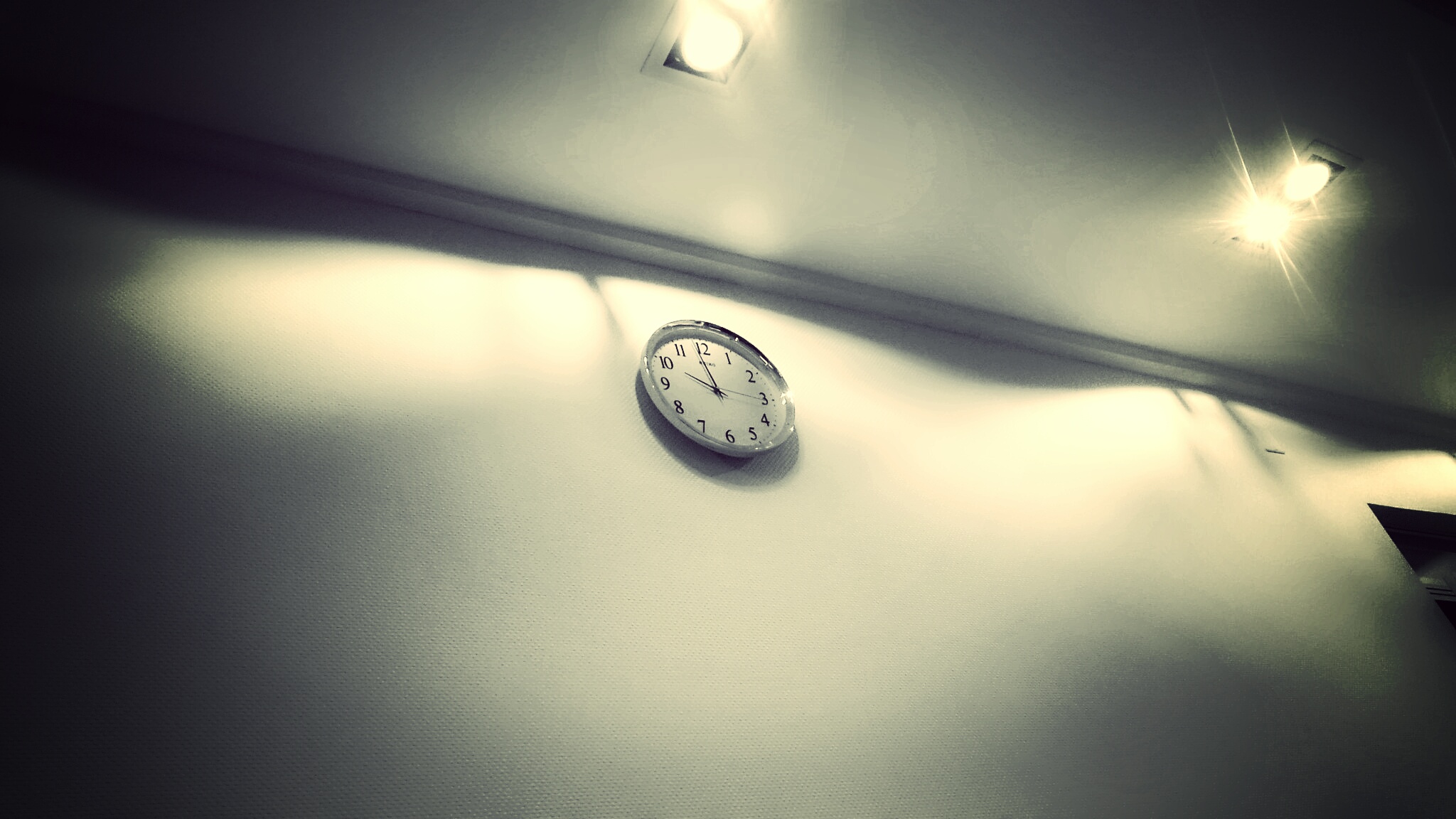This black-and-white photograph captures a simple office clock on a wall, evoking an almost eerie ambiance due to the stark lighting. The clock, with its chrome rim and white face bearing black numbers, is centrally positioned and indicates it is nearly 10 o'clock, with the second hand approaching the three. The scene is viewed from a low angle, as if the photographer were lying on the floor, looking upwards. Harsh ceiling lights illuminate the upper portion of the wall and cast strong shadows, highlighting the white molding where the wall meets the ceiling. Two visible light fixtures add to the high-contrast effect, one directly above the clock and another near the upper right corner. The rest of the room fades into darkness, save for a sliver of a door visible in the lower middle right corner, reinforcing the image's isolated and somewhat unsettling atmosphere.